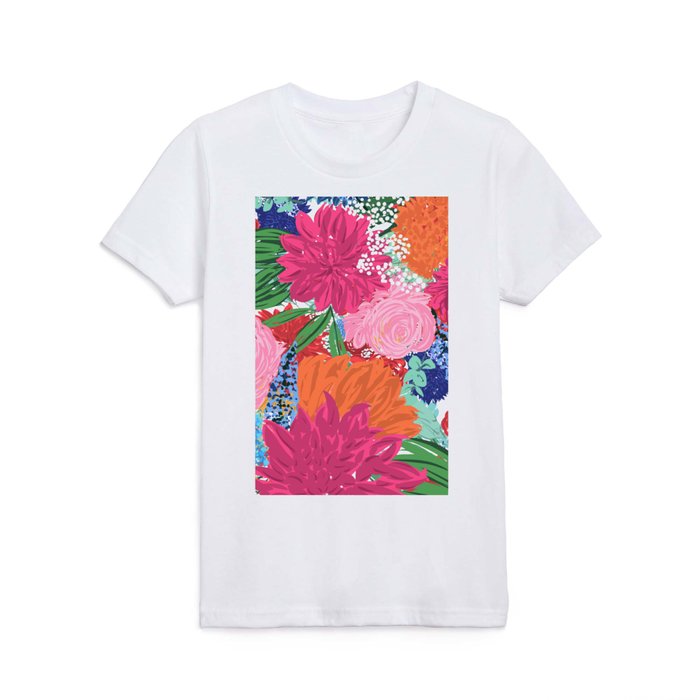This image features a short-sleeved, white cotton t-shirt with a scoop neck, laid flat on a white background. Dominating the center of the t-shirt is an impressionistic artwork of a bright and colorful flower arrangement contained within a vertically oriented rectangle. The floral design includes several types of flowers such as zinnias, roses, and possibly carnations, depicted in vibrant hues of pink, magenta, orange, pale blue, and white. Green leaves and stems add a touch of nature, along with white dots resembling baby's breath. The artwork appears painterly, with no text or logos visible, emphasizing the t-shirt's simple yet lively aesthetic. The t-shirt is displayed alone, highlighting its casual and informal style.